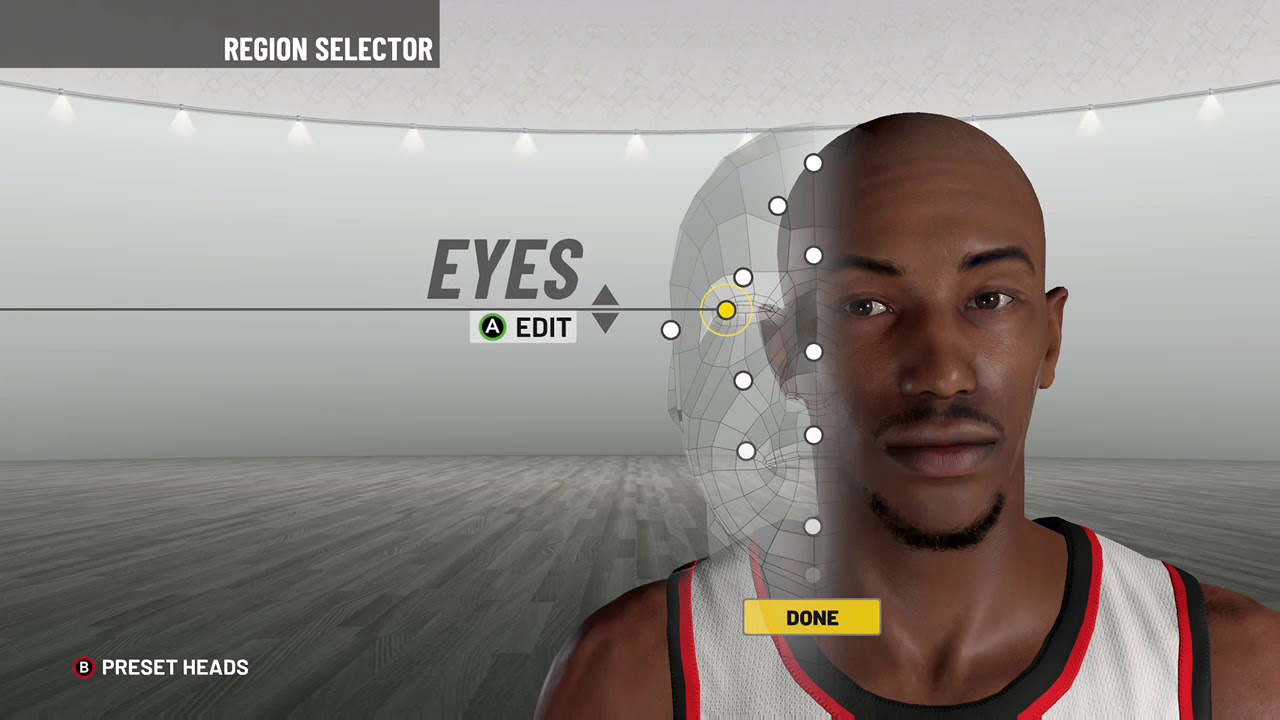This screen capture is from an NBA-themed basketball video game, specifically from the character customization menu. At the very top of the screen, "Region Selector" is displayed in white lettering within a dark gray box. The background features numerous spotlights and a gray wall with wood paneling or flooring beneath.

Centrally, the interface reads "Eyes," with options to "Edit" through designated "A" button prompts, including arrows for adjustments. A guiding line points towards the character's eye, indicating customization of eye shape or color. The featured character is an African American male, bald, with high-arched eyebrows, very dark eyes, a goatee, and smooth dark skin. He is dressed in a white, red, and black jersey, indicative of an NBA team.

Below the character, a yellow-boxed "Done" button is visible, followed by the label "Preset Heads" at the bottom of the screen.